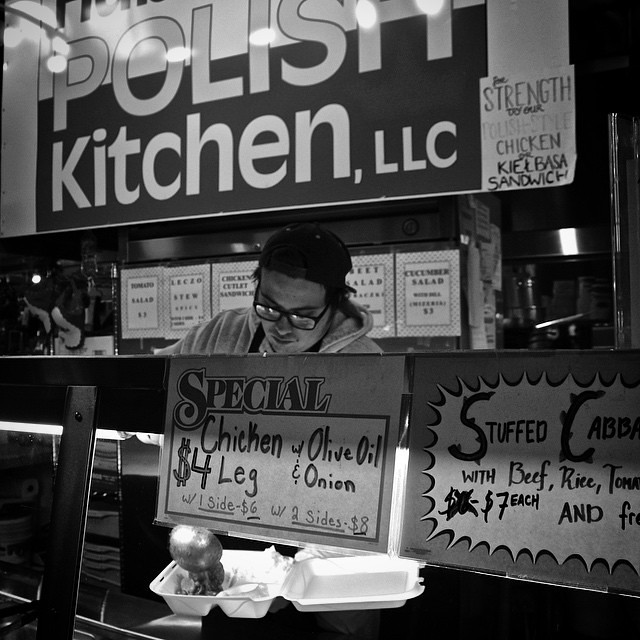This black and white photograph captures an old-fashioned kitchen setup, reminiscent of a takeout counter with a glass divider, much like one you might find at Chipotle. The top of the image prominently features a sign that reads "Polish Kitchen LLC." Below this, an employee, distinguishable by his glasses, backwards black baseball cap, and hoodie, is busy preparing an order. He is scooping food into an open styrofoam tray with a metal ladle. The prices and menu items, indicative of a bygone era, are clearly displayed on a sign affixed to the glass divider. The menu includes "special chicken with olive oil" priced at $4 per leg, $6 with one side, and $8 with two sides, and "stuffed cabbage with beef, rice, and tomato" at $7 each. Another sign invites customers to "Try Our Polish Style Chicken and Kielbasa Sandwich." The stark contrasts in the photograph add to the vintage feel of this bustling Polish kitchen.